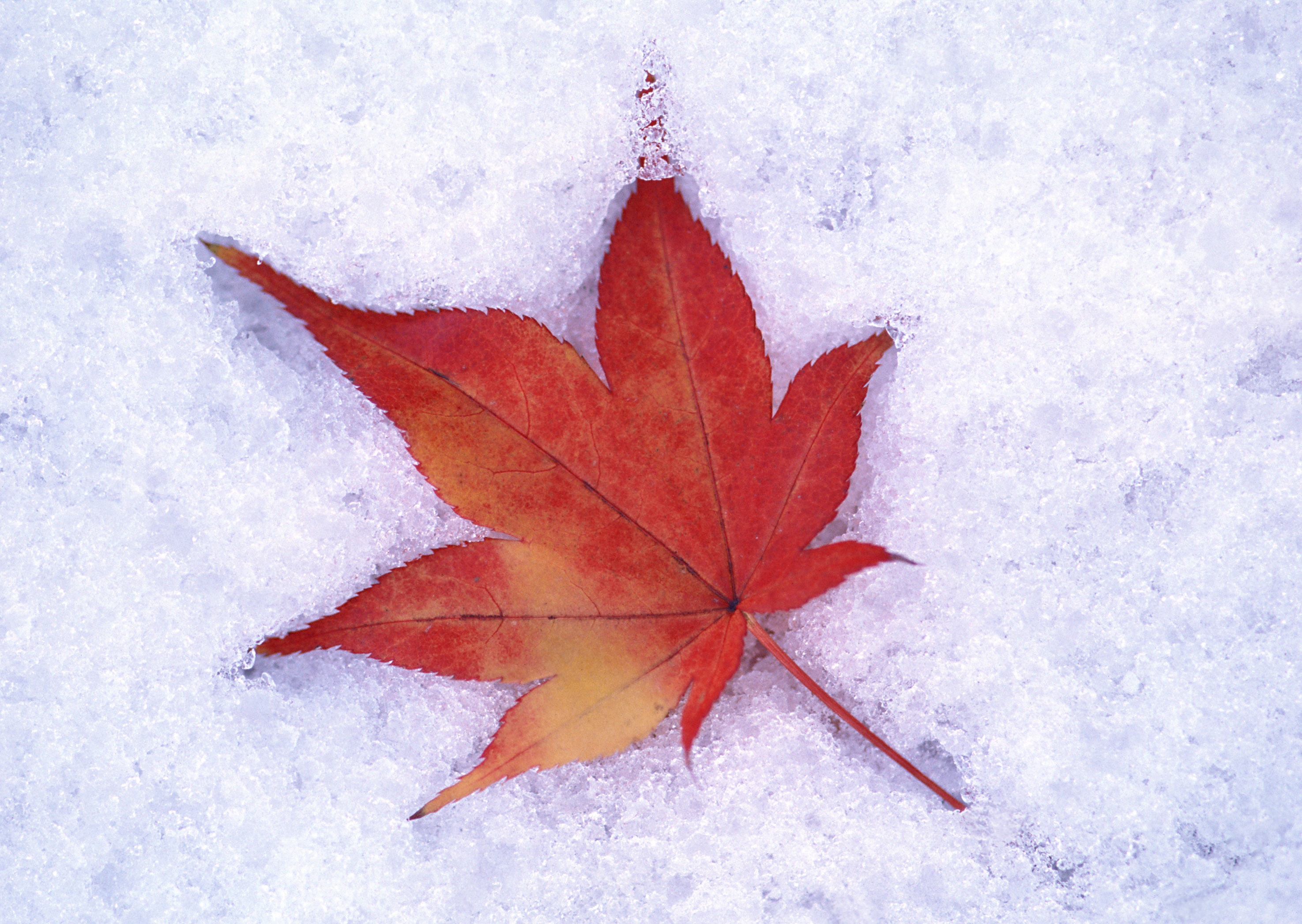In the image, a solitary leaf, predominantly red and transitioning to brown, lies on a soft bed of snow. The leaf, with seven deeply lobed, serrated fronds, displays intricate red veins. Its small red stem points towards the bottom right. Parts of the leaf are partially buried, with sections tucked under layers of snow and ice. The snow itself is a mix of soft, densely packed crystals, predominantly white with shades of bluish-gray, emphasizing the icy cold surroundings. A delicate print of the leaf is imprinted in the snow, outlining its contours and adding to the ephemeral beauty of the scene.